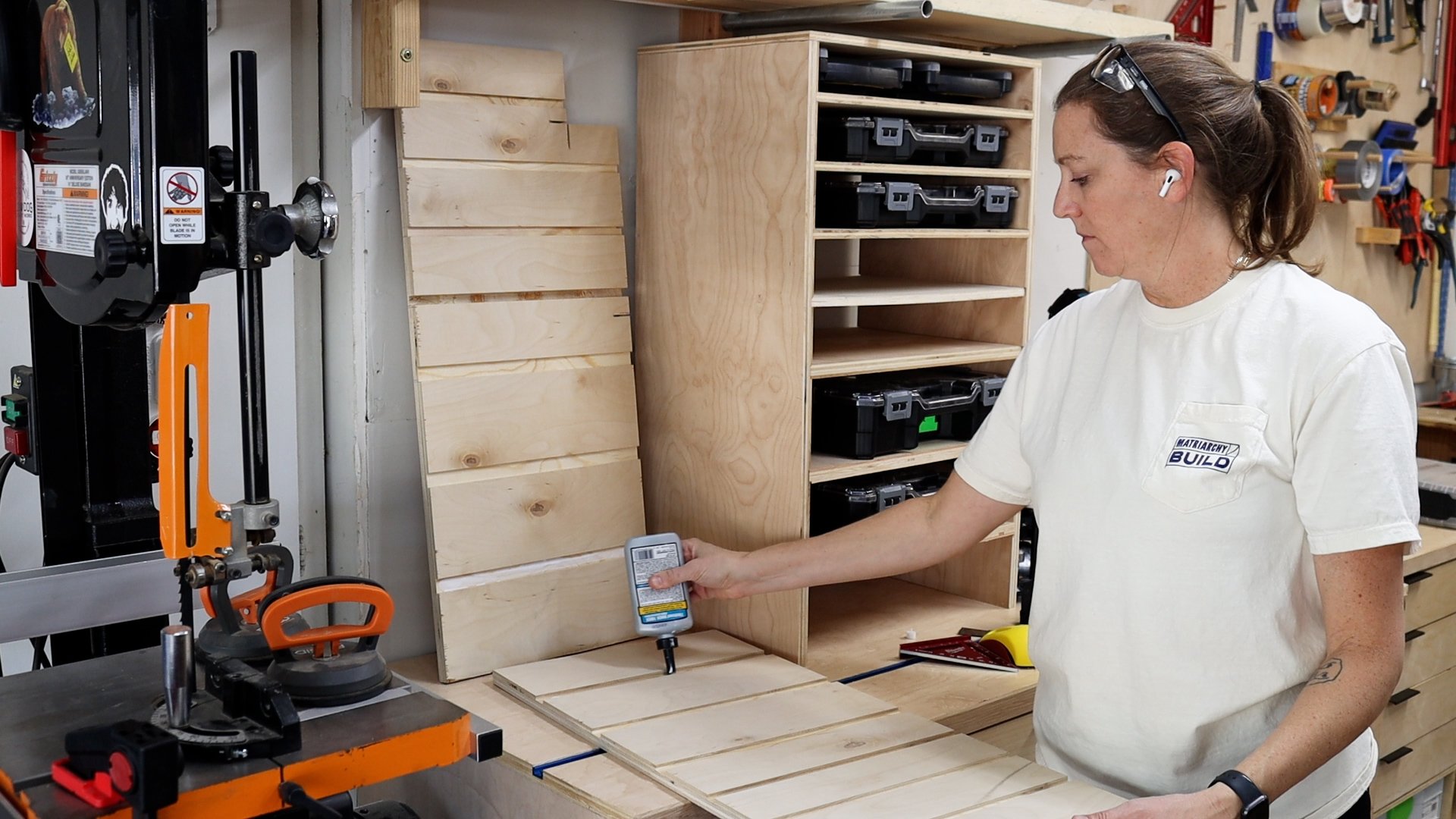In this detailed image, a woman is meticulously applying sealant or glue from a gray bottle into the divots of a wooden structure. She is dressed in a white t-shirt that reads "Build," signifying her association with a company. Her t-shirt has a pocket. Her hair is tied back in a ponytail and she has sunglasses resting on the top of her head and AirPods in her ears. She is light-skinned with brown hair and sports a tattoo on her left forearm along with a watch. Surrounding her work area are various wooden structures and a diverse array of tools. To her left, there is a sophisticated piece of equipment, likely a wood cutter or press, featuring orange and gray elements, with clamps in black, red, and orange. Safety signage is present on the machine, although it is unreadable from the image. Behind her are neatly organized toolboxes and a cabinet filled with multiple storage containers, as well as shelves stocked with additional power tools and materials, indicative of a well-equipped workspace.